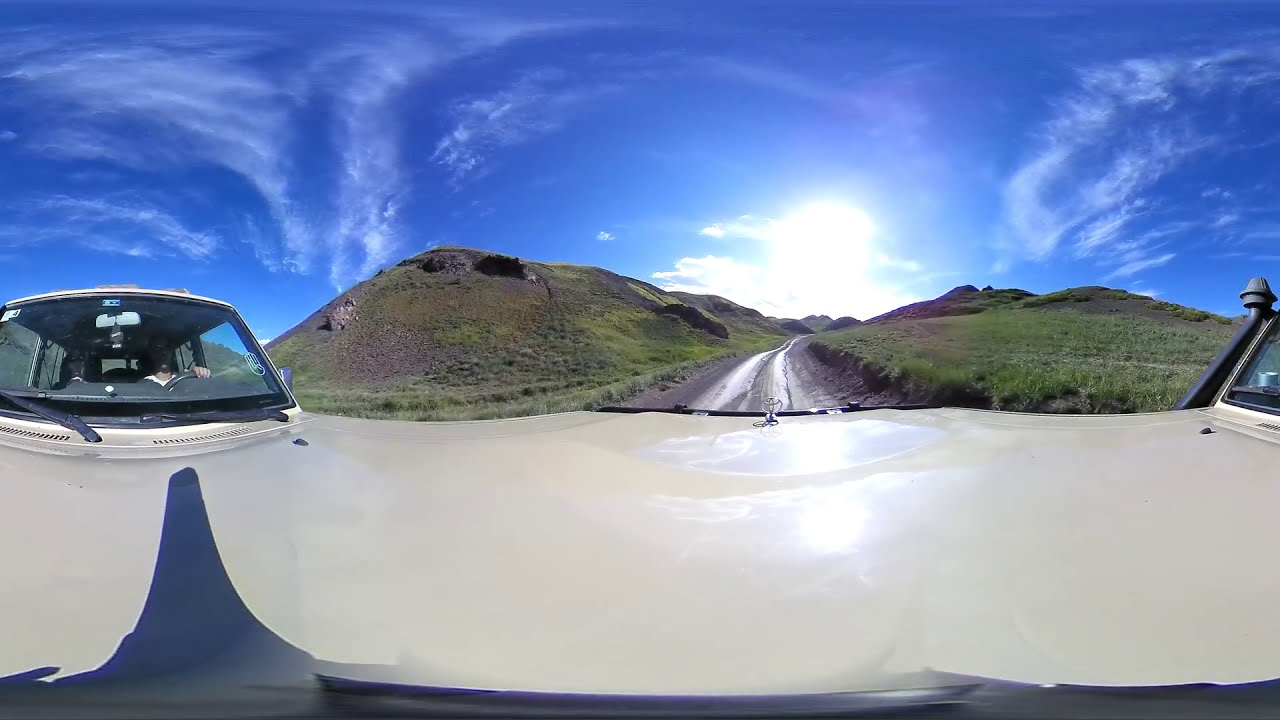The image captures a dynamic scene taken from a 360° GoPro camera mounted on the hood of a car. In the foreground, the distorted wide rectangular frame prominently features the metallic front of a white vehicle, stretching across the image and appearing on both the left and right sides. Visible through the windshield are a driver and a passenger. The road extends centrally through the photograph, seemingly a narrow mud path cutting through lush, gently rolling grassy hills. In the background, beneath a vibrant blue sky punctuated with wispy, soft white clouds, the sun casts a bright illumination over the landscape. The unusual camera angle and distortion create an intriguing, almost surreal duplication effect, adding a unique perspective to the scenic drive.